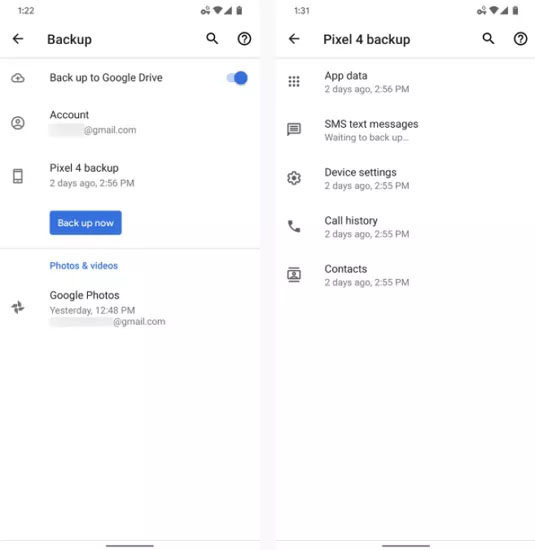The image displays two side-by-side screenshots, each occupying half of the total image width. 

The left screenshot, time-stamped at 1:22, features icons for Wi-Fi, phone service, and battery status at the top. This screenshot pertains to a Google Drive backup interface, highlighted with a blue tab that reads "Backup to Google Drive" next to a selection marker. Below are various options, including "Account," "Pixel 4 Backup," "Backup Now," "Photos and Videos," and "Google Phones."

The right screenshot, time-stamped at 1:31, shows the same icons for Wi-Fi, phone service, and battery at the top. It prominently displays "Pixel 4 Backup" and lists several backup options beneath: "App Data," "SMS Text Messaging," "Device Settings," "Call History," and "Contacts." The bottom two-thirds of both screenshots are entirely white, indicating the unselected or blank sections of each screenshot.